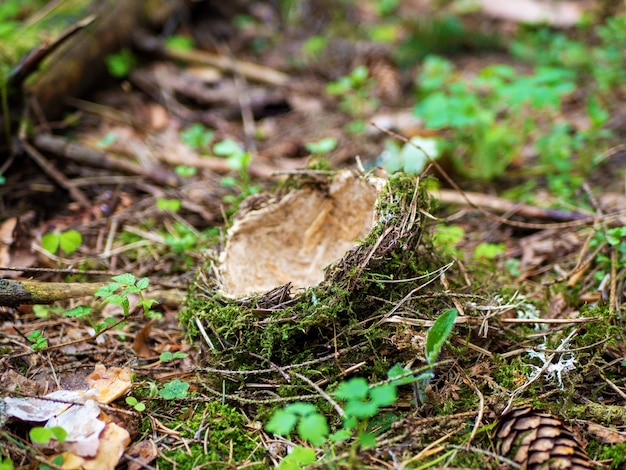This is a detailed, close-up color photograph capturing the forest floor, abundant with various natural elements. The vibrant green clover and small plants sprouting from the ground starkly contrast against the predominant backdrop of brown dead leaves, twigs, sticks, and branches scattered around. In the bottom right corner, a lone pine cone adds to the forest debris. Central to the photograph, commanding the viewer's attention, is an oval-shaped, half-dome object resembling a bird's nest or perhaps the shell of a large nut. This object is characterized by an exterior adorned with twigs and moss, giving it a somewhat hairy texture. The interior of this curious object reveals an off-white or lighter tan color. The image's composition directs a sharp focus on this central object, while the elements in the background fade into a soft blur, enhancing the depth of the scene and highlighting the natural lighting that bathes the forest floor.